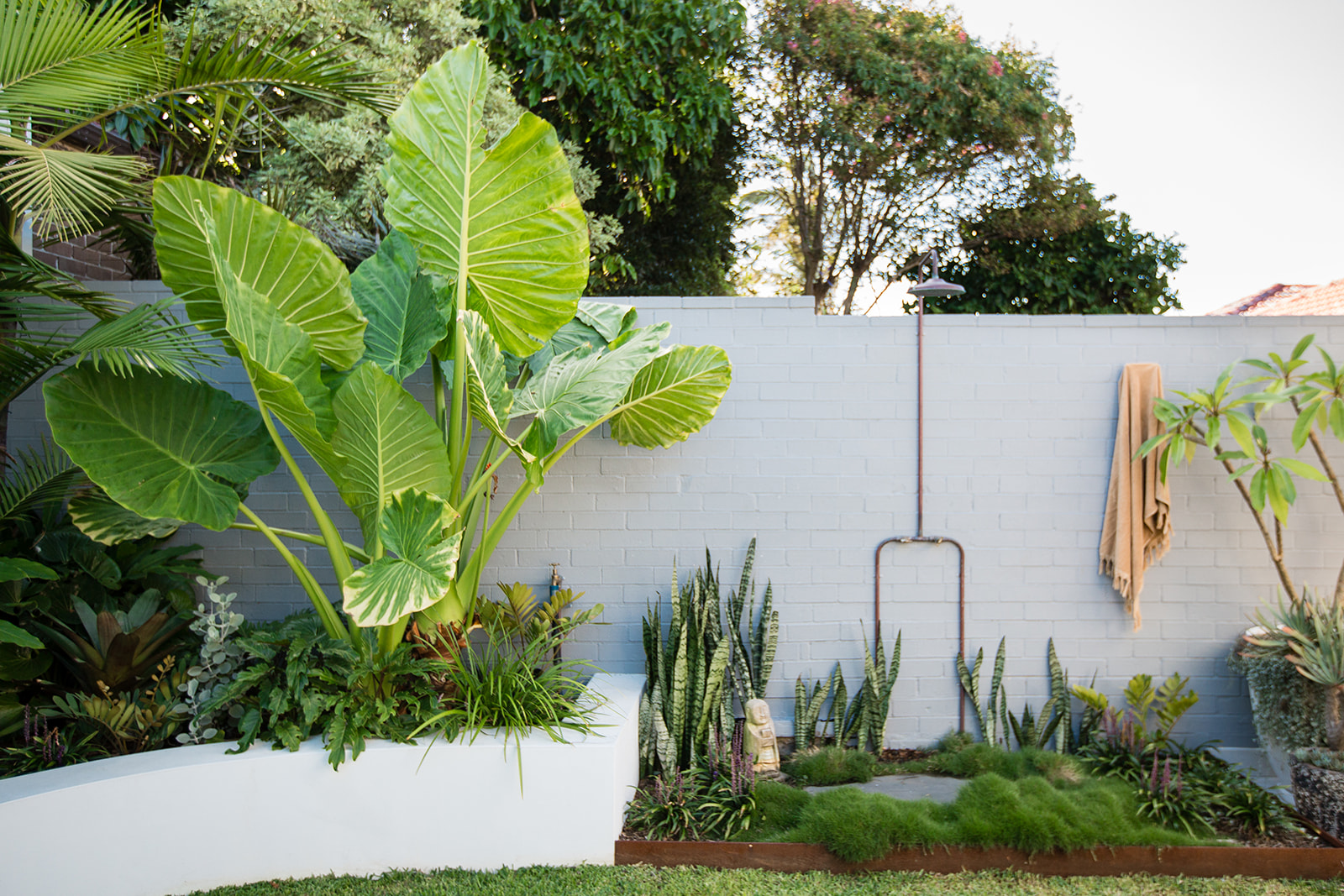This is a detailed garden scene captured in a backyard, showcasing a charming and lush landscape. Dominating the scene is a white brick wall stretching across the image. In the top right-hand corner, a sliver of a clear sky—either white or very light blue—is visible. The upper portion of the image is framed by thick trees, primarily on the left side, thinning out toward the middle to reveal some striking purple blooms among the foliage.

The center of the image features a varied collection of plants within a raised white flower bed that extends from the center to the left edge. This bed hosts a diverse array of flora, including small, stringy green plants, red plants, a couple of light blue plants, and a notably large plant with long stems and gigantic leaves. Nestled among these plants are tall aloe specimens, surrounded by small green bushes and occasional red leaves.

In the middle of the photograph, centered against the white wall, stands a small Buddha statue beside a serene, moss-bordered pond. A metal pipe, or bracket, extends from the top of the wall, looping into a U-shape above the pond area. Adjacent to this serene setup, on the solid white wall's far right side, a peach-colored quilt or towel hangs nonchalantly. The base of the image shows a white curb jutting out from the wall, in front of which lush grass is thriving, enhancing the garden's vibrant appeal.

Additionally, thin-branched green plants are seen on the right side, with what looks like water from a small fountain spraying in the air nearby. The background features more high trees with palm leaves peeking over, belonging to the neighboring property, completing this picturesque and tranquil garden scene.